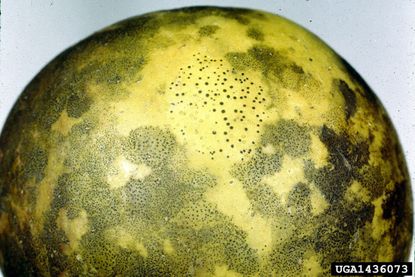The image depicts a spherical, yellowish-green object resembling a moldy lemon or lime, with uneven coloration across its surface. Dark green and light yellow areas are scattered unevenly, with clusters of black speckles concentrated primarily on the top. The background is a light teal color, providing contrast to the sphere. In the bottom right corner, there is a black rectangle with an identification number, "UGA 1436073."